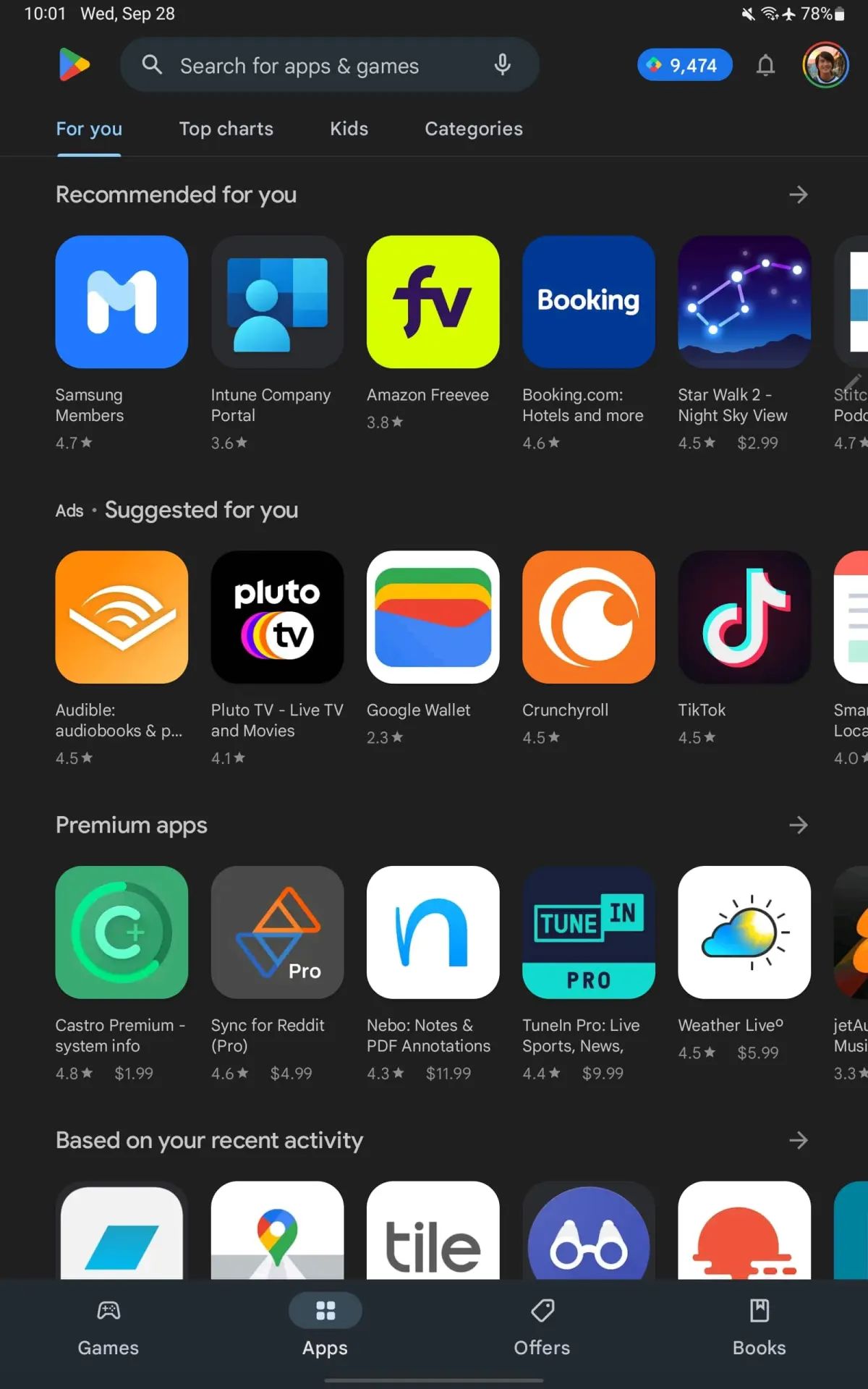This image captures a detailed view of the Google Play Store interface. At the top left, the screen displays the Google Play logo and a text reading "Google Play." The device status bar at the top right shows the time as 10:01 on Wednesday, September 28th, along with Wi-Fi connectivity and battery percentage indicators.

Below the Google Play logo, there's a prominent search box. Next to it, a blue number reads "9,474," likely indicating available updates or notifications. Adjacent to this is a notification icon and the user's profile icon. 

The interface highlights the "For you" tab, among other tabs such as "Top charts," "Kids," and "Categories." Under the "Recommended for You" section, several apps are listed including Samsung Members, Intune Company Portal, Amazon Preview, Booking.com Hotels & More, Star Trek 2, Night Skyview, and Ads Suggested for You like Audible and Food Lord TV. Other suggested apps include Live TV, Google Wallet, Crunchyroll, Tik Tok, Premium Apps, Castro Premium System Info, Sync for Reddit Pro, Nemo Notes and PDF Annotation, Totals Pro, and Live Sports, News, Weather Live. The section based on recent activity includes app suggestions, although the titles are illegible.

At the bottom of the screen, four primary navigation tabs are visible: Games, Apps, Offers, and Books, allowing quick access to different sections of the store.